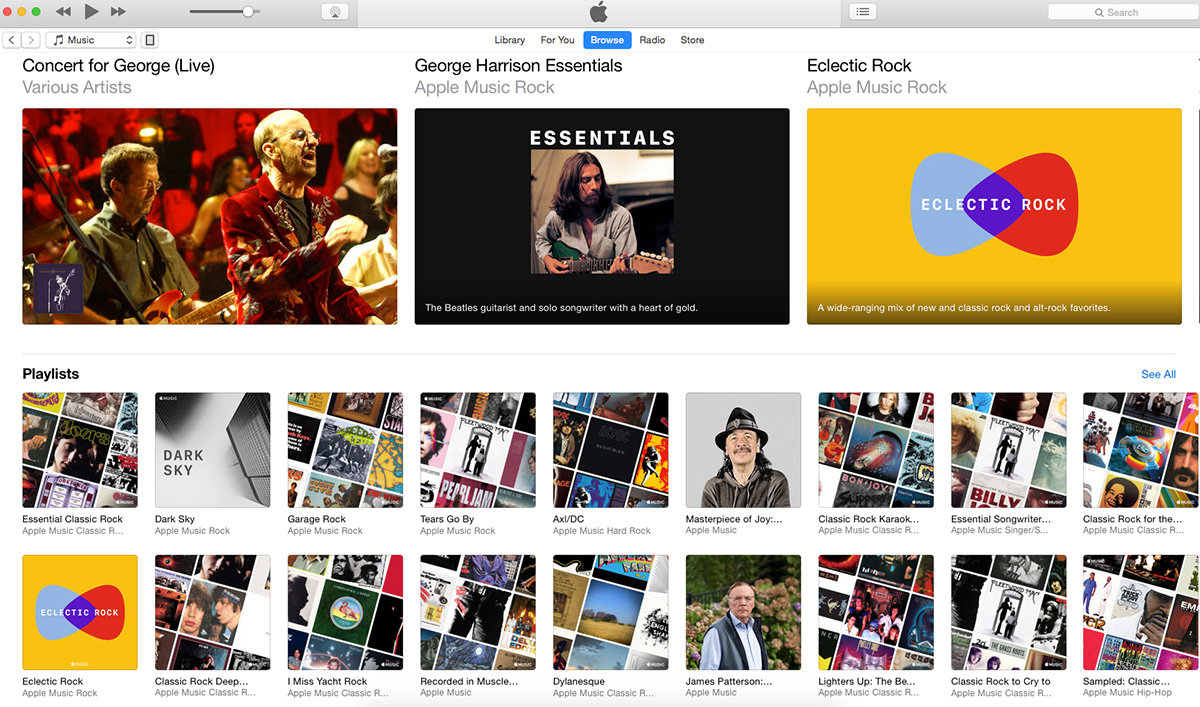The image displays the iTunes interface prominently featuring the Apple logo at the very top. The interface has a gray theme with red, yellow, and green buttons located in the top-left corner. Key navigation controls such as the play button, backward button, forward button, and a search bar are found towards the top right.

Under the primary navigation bar, options including "Library," "For You," "Browse," "Radio," and "Store" are visible, with "Browse" highlighted in blue. Below this, there are several clickable sections.

The first segment features "Concert for George: Live" by Various Artists, accompanied by an image of a man in a red suit singing, alongside another individual playing the guitar.

The next section showcases "George Harrison Essentials" under the Apple Music Rock category. The visual portrays a black-themed cover with the word "Essentials" and a photo of a man playing a guitar. This segment highlights "The Beatles guitarist and solo songwriter with a heart of gold."

Following this, "Eclectic Rock" under Apple Music Rock is displayed. It features a design with two pick-like graphics and a description stating "A wide-ranging mix of new and classic rock and alt-rock favorites."

Below these sections, there's a "Playlists" area displaying multiple thumbnails representing various album collections.